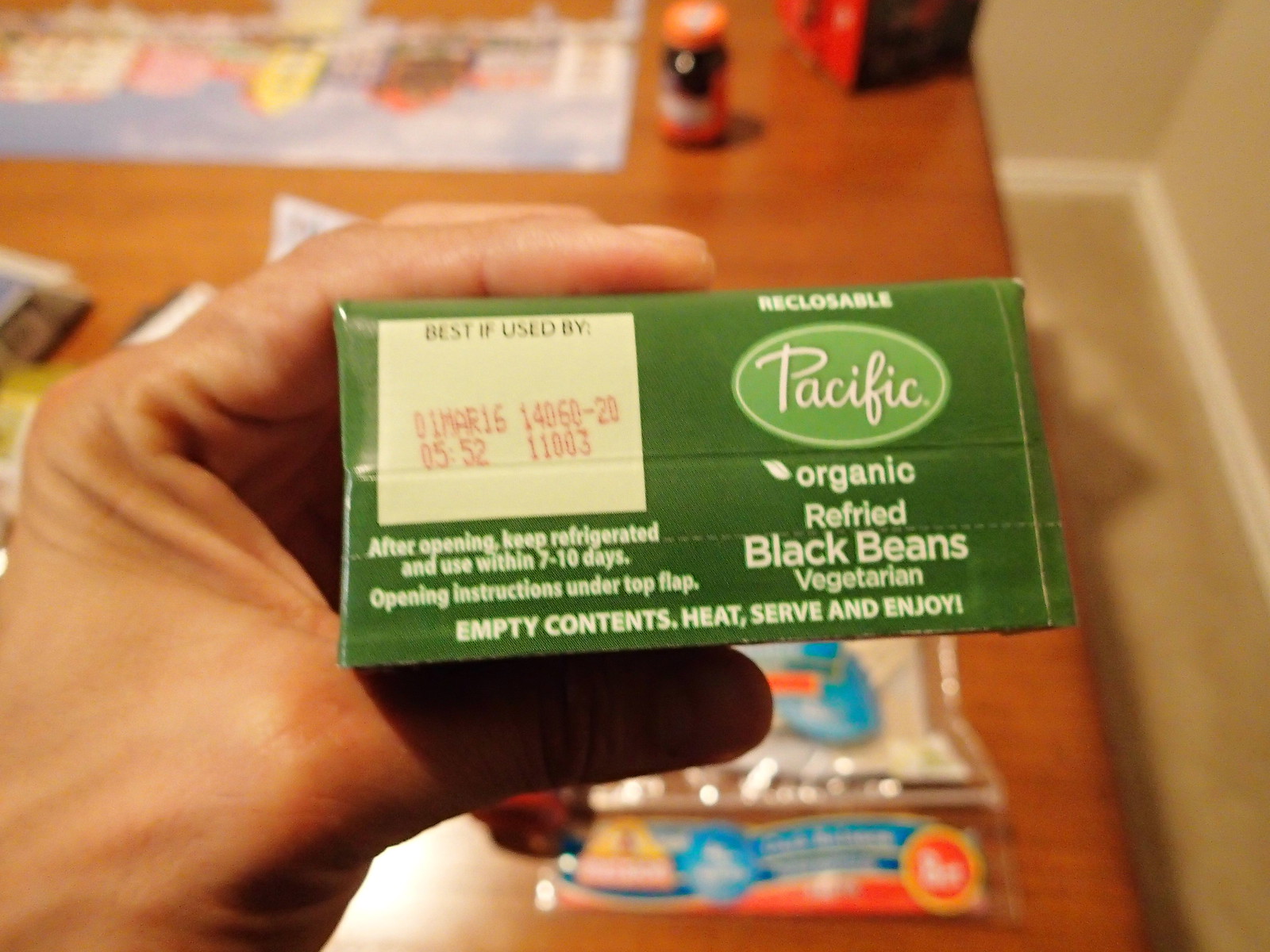In this photograph, a left hand is prominently holding a box of Pacific brand organic refried black beans, which are vegetarian. The hand is positioned with fingers on top and the thumb below the package, presenting the box to the viewer. The brand name "Pacific" is displayed in an oval-shaped, light green logo in the upper right-hand corner. Above the logo, the word "recloseable" is printed. On the upper left-hand side, there is a white box indicating the best-by date, which reads "01 MAR 16" followed by the codes "1460-20, 05:52, 11003".

The packaging is green and provides additional instructions: "After opening keep refrigerated and use within 7-10 days. Opening instructions under flap. Empty contents. Heat, serve, and enjoy!" In the background, a fuzzy image of another package rests on a brown table, along with a glimpse of tan flooring to the right. The detailed setup suggests a well-used kitchen space.